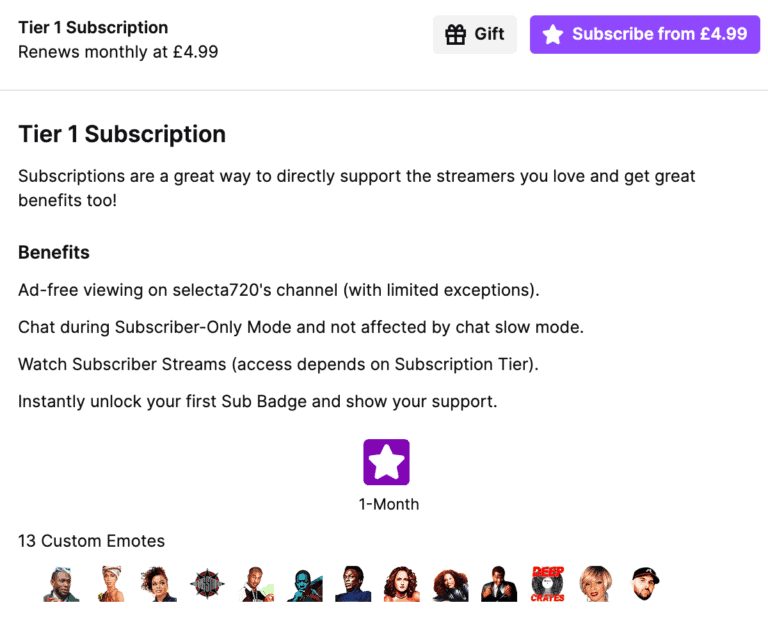In this image, the interface resembles a subscription page. At the top right, there's a rectangular box with a purple background that says "Subscribe from £4.99," and to the left of this text is a white star. Further left, there's a smaller rectangular box labeled "Gift," accompanied by a black present icon.

In the top left corner, the text "Tier 1 Subscription, renews monthly at £4.99" is displayed. A line separates this section from the next.

In the second section, the header reads "Tier 1 Subscription." Below it, the text explains that subscriptions are a great way to directly support the streams you love while earning great benefits. The term "Benefits" is bolded, followed by details: ad-free viewing on Selective720's channel with limited exceptions, chat during subscriber-only mode without slow chat restrictions, watch subscriber streams, and instantly unlock your first badge to show your support. An icon of a one-month badge is also pictured.

At the bottom left, there's text stating "13 custom emotes," accompanied by a variety of small emoticon icons.